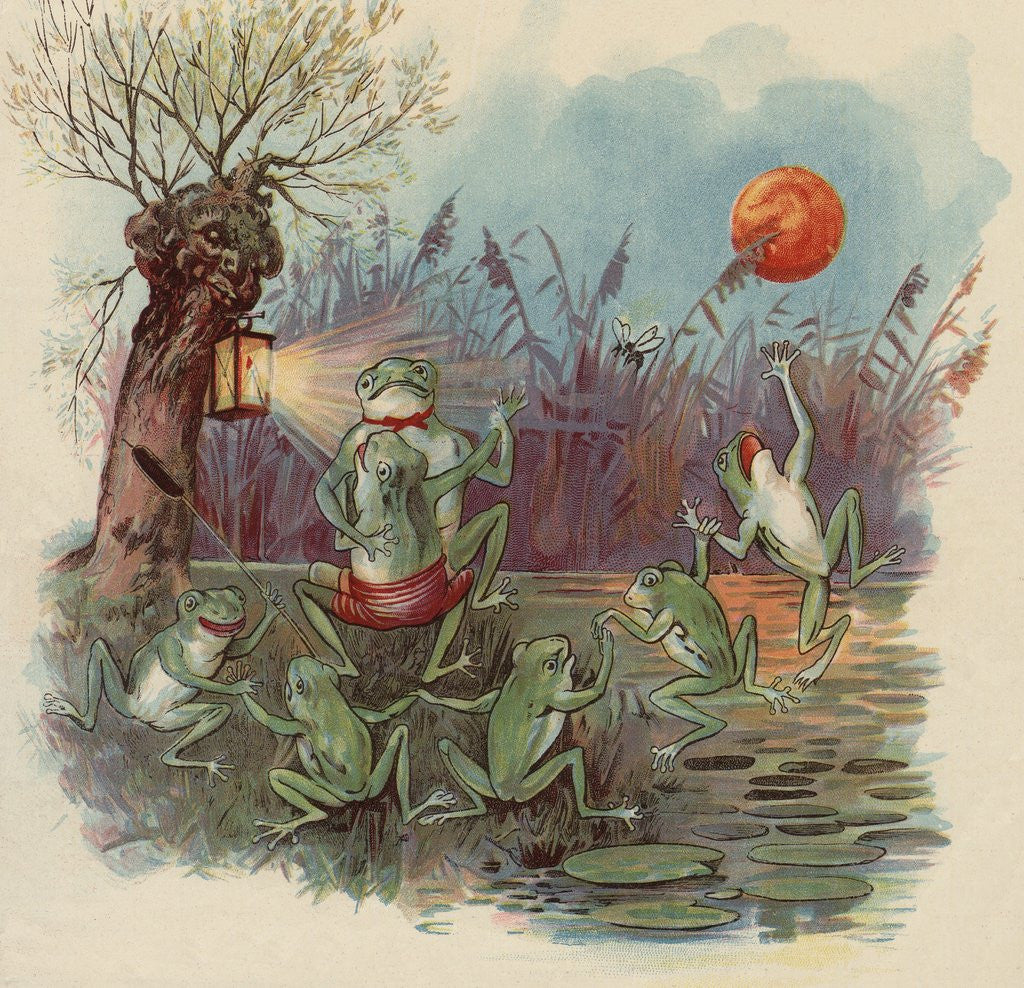In this detailed painting on canvas, a whimsical scene unfolds in a vibrant swamp under an evening sky illuminated by an orange glow. At the center is a joyous line of five cartoonish frogs, standing on their hind legs and holding hands as they dance merrily. One frog on the left clutches a cattail, while the frog furthest to the right leaps upward, seemingly aiming for a floating orange ball above. Behind this line, a couple of frogs dance intimately; the male wears a red bow tie and the female is adorned in red and white shorts. A lantern hangs from a nearby tree with a face carved into its trunk, casting beams of light over the dancers and highlighting the scene with an enchanting glow. Above the frogs on the right side, a fly buzzes around near a foreboding blood-red moon. The picturesque setting includes lily pads floating on sparkling water, adding to the magical atmosphere of this enchanting swamp.